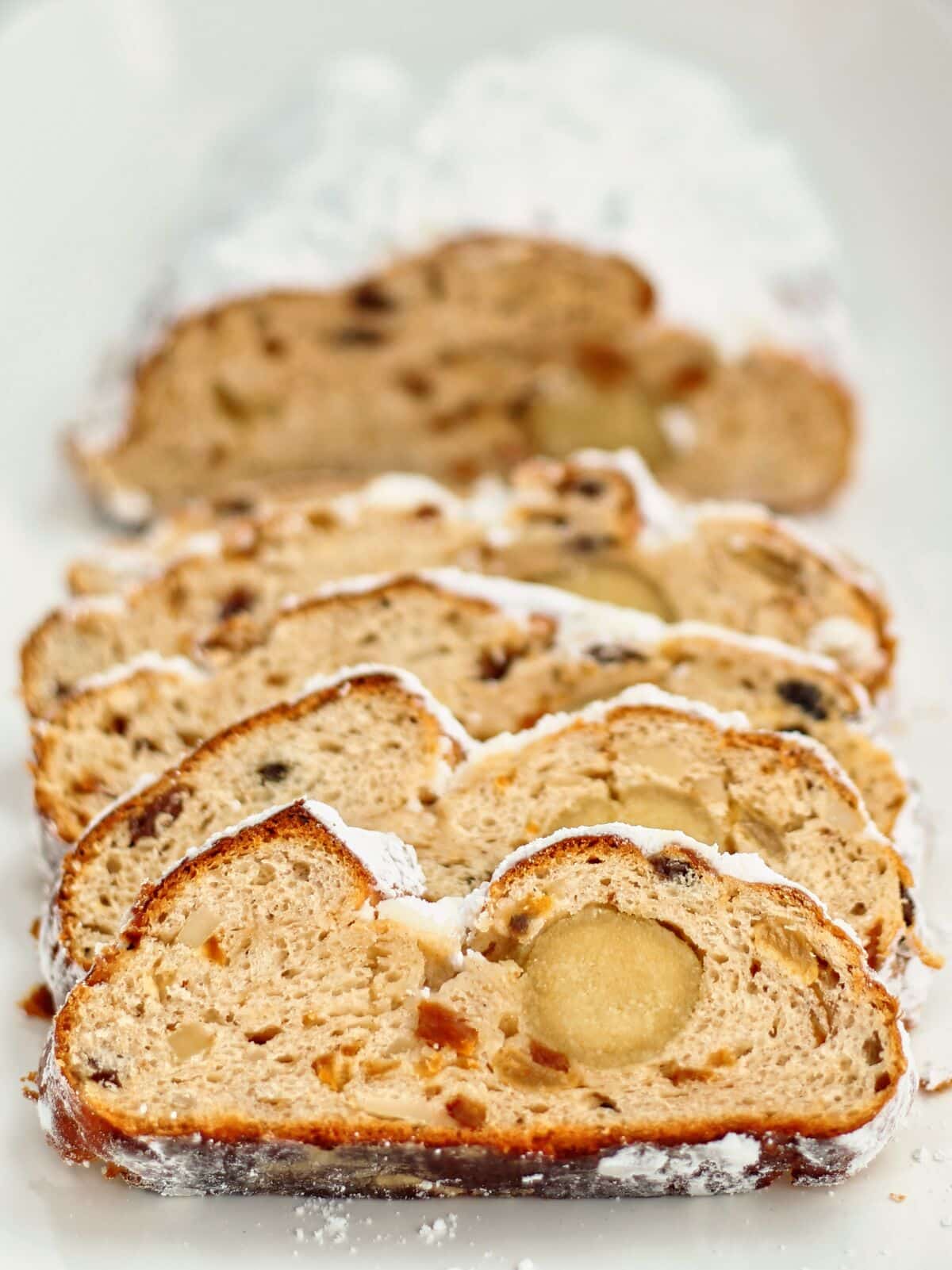This is a photograph of a fruit loaf, resembling a fruit cake. Half of the loaf has been neatly sliced, with four slices arranged in a domino-like fashion in the foreground. These colorful slices reveal bits of dried fruit, with hues of red, yellow, brown, and green. The bread has a dark brown crust generously coated with powdered sugar, which also covers the top and bottom of the uncut portion in the background. The entire setup rests on a white surface that resembles a tablecloth, enhancing the visual appeal of the white powdered sugar against the backdrop.